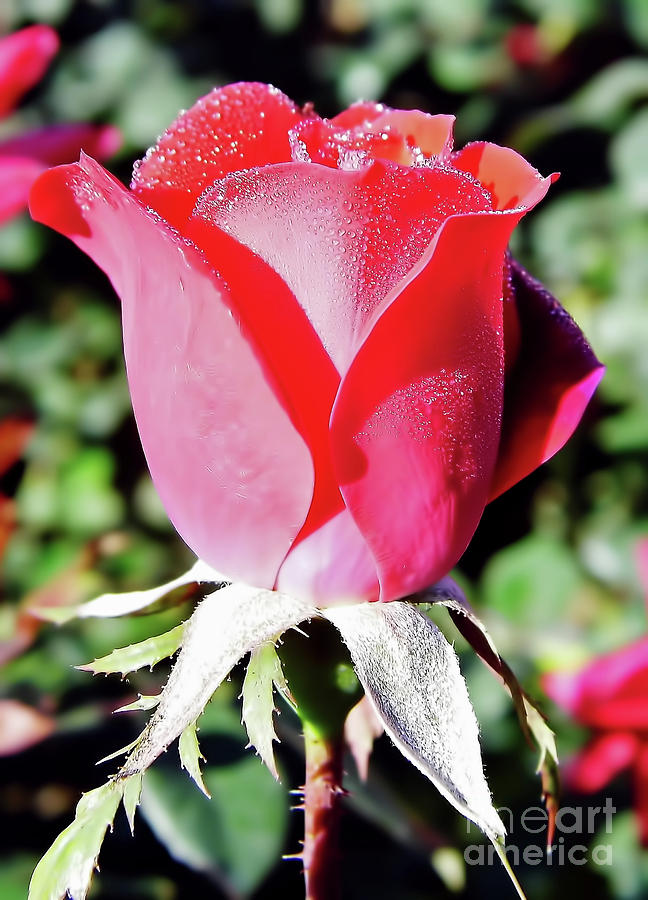This is an extremely detailed close-up photograph of a single, deep pink rose that is in the process of blooming. The composition focuses mainly on the rose bud, which fills most of the frame. The petals are slightly open, standing upright and covered with glistening droplets of dew, adding a sparkling effect to the flower. At the base of the petals, there are small green leaves spreading outwards, and the green stem transitions into a darker reddish-brown color as it descends. The background features blurred foliage and greenery, interspersed with out-of-focus hints of other roses, emphasizing the primary subject of the image. The overall effect is a vivid and beautiful depiction of a single rose with a moist, radiant allure against a backdrop of verdant surroundings.